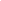This detailed, science fiction fantasy illustration depicts two muscular, mechanical warriors clad in elaborate armor. The dominant figure in the foreground on the left stands out vividly with its striking red metal helmet adorned with six circular elements arranged in three pairs. Its imposing armor features a black breastplate, embellished with yellow and golden ornaments, and prominent red shoulder plates. The second warrior, slightly obscured and hazy to the right, mimics the first in design, sporting a similarly shaped helmet and armor. This figure wields a large staff or trident-like weapon with a glowing purple sphere at its tip. The backdrop consists of a sky filled with black and white clouds, dotted with stars, under a light blue expanse, adding to the fantastical atmosphere of the scene.